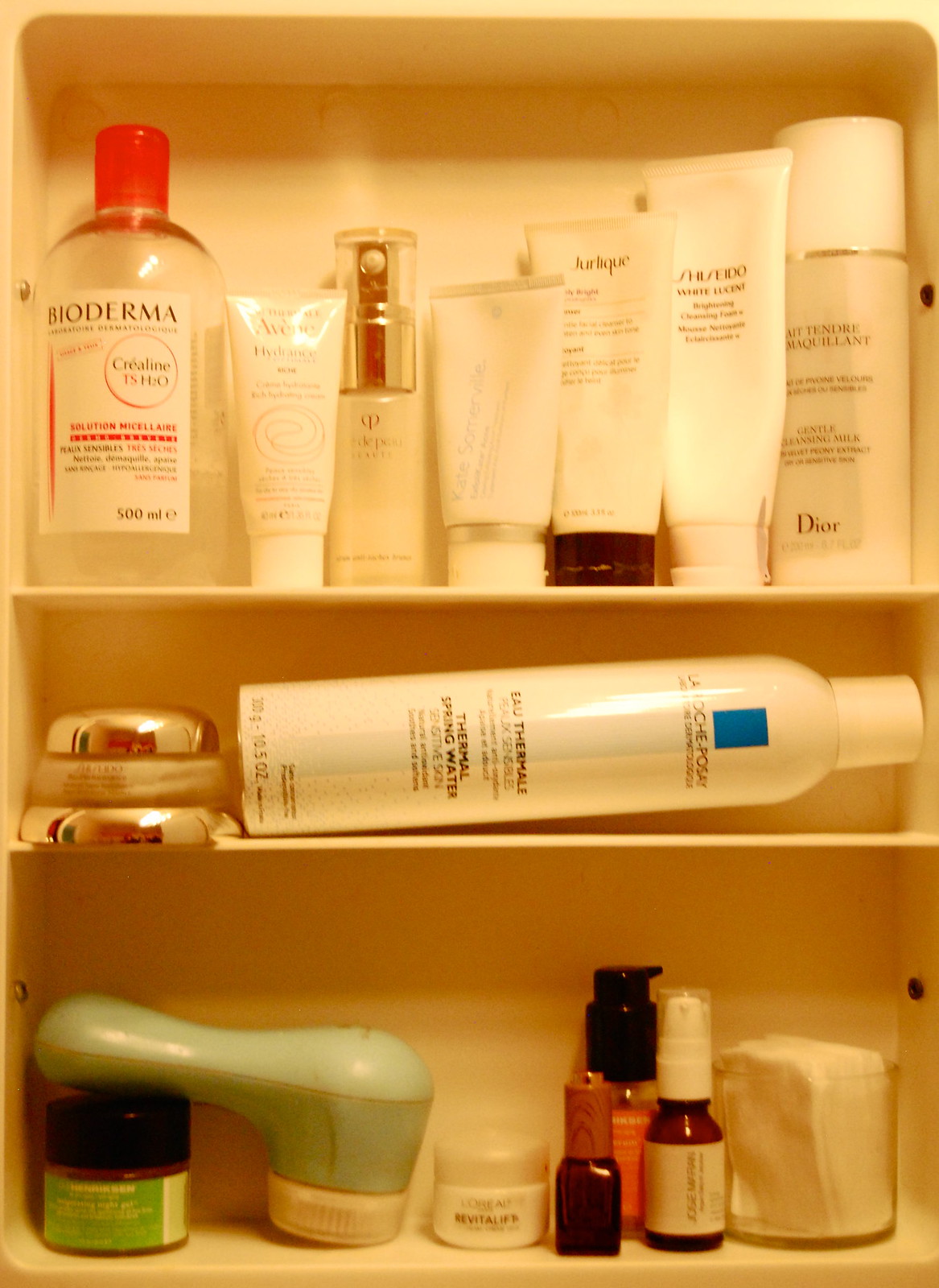This close-up photo showcases the interior of a recessed medicine cabinet attached to a wall. Noticeably, the cabinet lacks a door and features three shelves encased in a plastic frame with a yellowish hue. The top shelf, being the tallest and most spacious, holds a variety of seven items. These items include four tubes which likely contain hand cream or face cream. Among them is a small bottle labeled "Bioderma," filled with a white liquid and sealed with a red cap. Additionally, there is a small bottle equipped with a spray top, suggesting it could be a perfume or cologne. On the far right sits a plastic jar topped with a white cap.

The middle shelf, narrower in size, contains a horizontally placed white bottle with a blue rectangular label and the words "Thermal Spring Water" visible on the front. This bottle, capped in white, rests against the right edge of the cabinet. Adjacent to it, on the left side, is a highly reflective golden metallic object, which appears to be a case for an unknown item.

The bottom shelf is filled with a diverse assortment of products. Among them are some cotton pads and an antique-looking device resembling a tiny hair dryer, encased in green. Positioned under the handle of this device is a wide jar, while to the right are several bottles. These include a short, squat white bottle and two or three glass containers, one of which features a spray attachment on top.